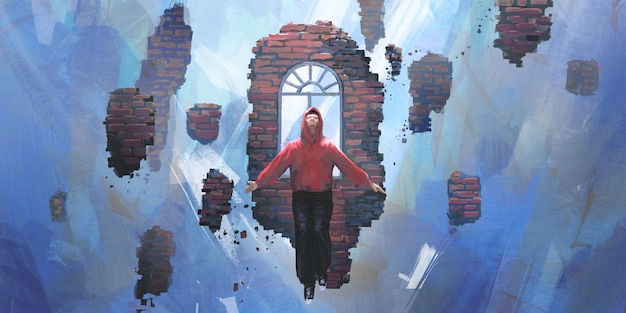The image portrays a striking artistic scene where a young Asian man, clad in a bright red hoodie with the hood up, dark pants, and black Converse shoes, appears to be bursting out of a brick wall. The dynamic moment captures him in mid-air, arms extended diagonally, head tilted upward, giving the impression of levitation or flight. The force of his breakthrough sends bricks flying outward in all directions, emphasizing the dramatic explosion of the wall. Just behind him, an arched window remains intact amidst the chaos, mounted within the remnants of the brick wall. The background, featuring abstract light blue and white hues, along with hints of cliff sides, enhances the ethereal quality of the scene, blending realism and surrealism beautifully.